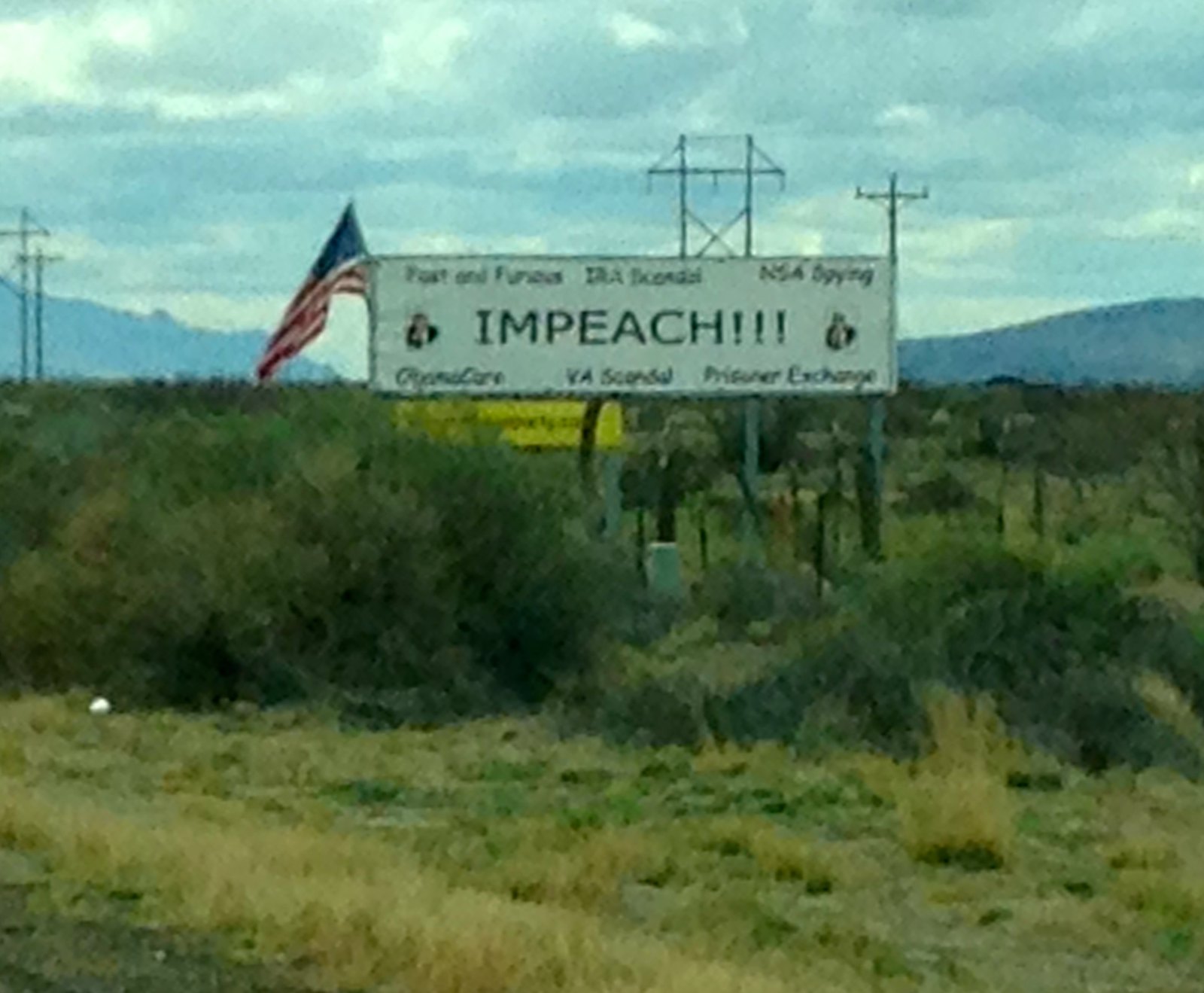The photograph captures a large, white rectangular sign positioned prominently in a rural, almost desert-like area with mountains faintly visible in the background. The sign is mounted on wooden posts and features an American flag hanging from its top left side. The text on the sign is a call for impeachment, boldly stating "IMPEACH!!!" along with reasons scattered across it, such as "VA Scandal" and "Prisoner Exchange." Additional phrases like "Fast and Furious" and "NSA" are noted, although some text remains illegible due to the distance and blurriness of the image. The background includes tall power lines with an H-shaped structure, under a cloudy sky. The foreground is marked by scruffy yellowed bushes and patches of green grass.